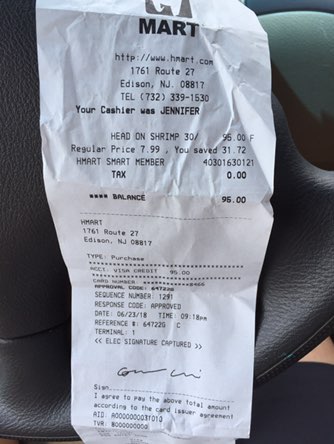A detailed photograph depicting a receipt positioned on a dark gray steering wheel. In the lower part of the image, a person's leg is visible, showing partial skin and dark-colored shorts. The receipt, marked in black at the top, displays an address at 1761 Route 27, Edison, New Jersey, along with a phone number (732-339-1530). It indicates that the cashier's name was Jennifer. The transaction includes a significant purchase of shrimp for $95. Additional details include a service member number, a response code, and the date of June 23, 2018. The time of the transaction is also listed. At the bottom of the receipt, there is a handwritten signature.